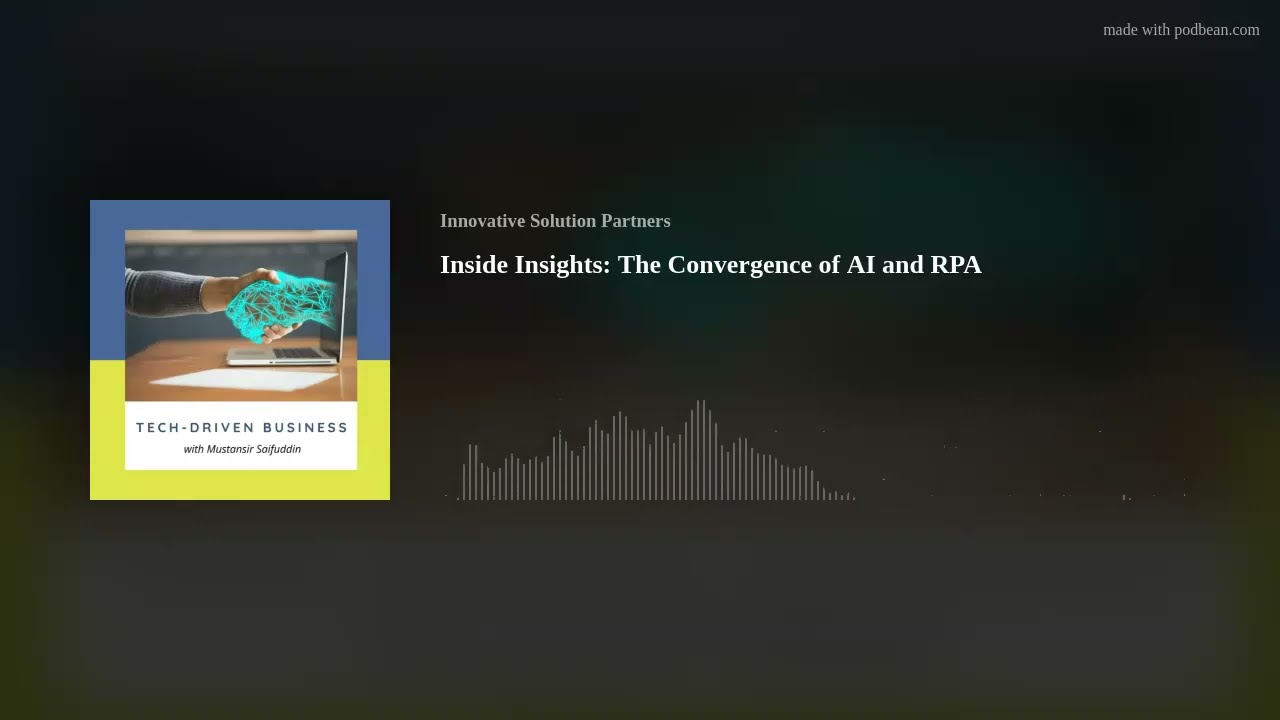The image is a detailed promotional slide for a tech-driven business presentation or podcast. The background is black with a small white text in the top right corner that reads "Made with Podbeam.com." On the left side, there's a rectangular image framed by a blue top border and a yellow bottom border. This image depicts a hand emerging from a laptop, made of blue wireframe lines, shaking a human hand. Above and below this image, which appears to be part of the cover art or main visual, are separated by color blocks: the upper is blue and the lower yellow. In a white box beneath the image, the text reads "Tech Driven Business by Mustafar Sufadan." 

To the right of this visual, the main content text states "Innovative Solution Partners, Inside Insights: The Convergence of AI and RPA," accompanied by a bar graph graphic in white font below. The overall design integrates various elements to convey a message about the intersection of artificial intelligence (AI) and robotic process automation (RPA).